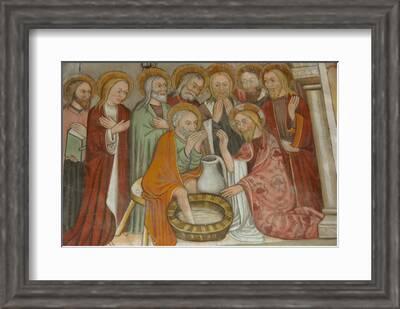This image features a dark gray-framed picture with a white inlay canvas creating a border around the artwork. The scene appears to depict a religious ceremony, possibly a depiction of Christ washing the feet of an apostle. At the center of the image sits a man with gray hair and a beard, dressed in an orange-yellow robe, with a halo above his head, indicative of enlightened or holy status. This man has his right foot dipped into a brown basin filled with water. Situated to his right is another man, identified by his red robe and the act of blessing the man in the basin, who also has a halo around his head, suggesting he may be Christ. Between them sits a white ceramic pitcher, possibly used for the foot-washing ritual.

Surrounding these central figures are seven other individuals, all adorned in various colored robes—primarily red, light green, and yellowish-orange—and each with a halo, suggesting their holy nature. Some of these figures hold books and have their hands clasped in a prayerful fashion, emphasizing the religious context of the scene. The background includes a white marble arch on the right, enhancing the sacred atmosphere of the setting. The entire image conveys a solemn, ceremonial event with strong religious undertones.